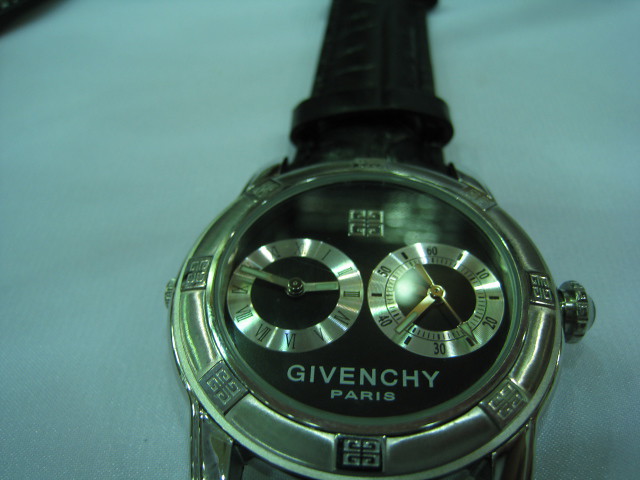This detailed close-up image showcases the face of a Givenchy Paris watch, prominently centered in the frame. The overall tone of the photograph leans towards a cool, greenish hue, likely influenced by the ambient lighting. The watch face is set against a light-colored background, which subtly contrasts with the intricate details of the timepiece.

The bottom edge of the watch face aligns precisely with the bottom of the image, concealing the lower watch strap from view. The upper strap, however, is partially visible, featuring a sleek silver metallic frame. The watch face itself is sophisticated, adorned with two sub-dials and circles.

Interestingly, the sub-dial on the left displays Roman numerals, while its counterpart on the right uses Arabic numerals. These sub-dials present different times, adding a layer of complexity to the timepiece. Clearly printed on the bottom of the watch face, just above the frame, is the brand name "Givenchy Paris," affirming the luxury and elegance of this watch.